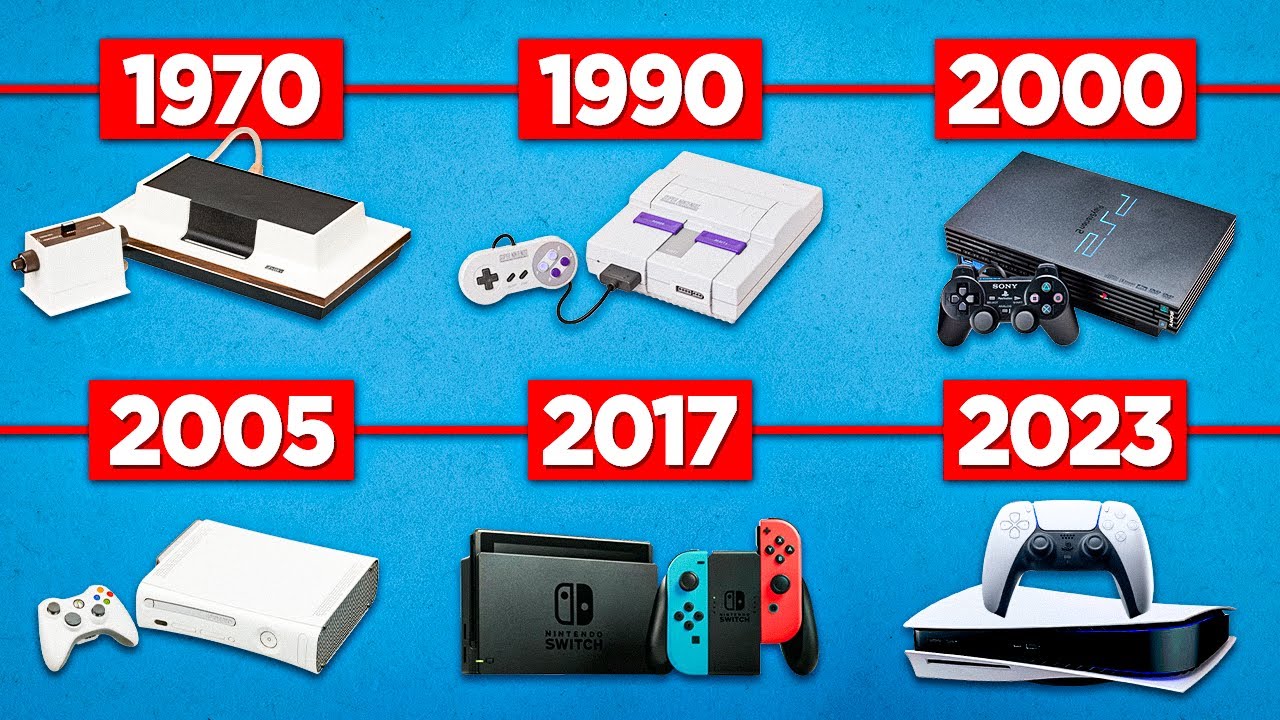The image is a detailed timeline displaying the evolution of video game consoles from 1970 to 2023. The background is blue, and the years and connecting lines are in white font set against red boxes and lines. The years and their corresponding consoles are arranged in a 3x2 grid format. 

- **1970**: Exhibits an Atari 2700, a long, rectangular white console with a black top. The controller, resembling an electric pencil sharpener, is white with a black button on top and a knob on the left.
- **1990**: Features a Nintendo NES, a white console with two purple buttons on the top. The controller is connected to the left port.
- **2000**: Displays a PlayStation 2, a sleek black rectangular console with "PS2" in blue. The controller is propped against the front.
- **2005**: Shows an Xbox 360, white and positioned on its side with visible metallic grating. The wireless controller lies beside it.
- **2017**: Highlights a Nintendo Switch, a compact black console with "Nintendo Switch" on the front. The controller features detachable sides, one turquoise blue and the other red.
- **2023**: Contains a PlayStation 5, a modern, futuristic console with a black center and white exterior, laying on its side. The controller, also in black and white, is perched atop the console.

The image visually emphasizes the technological and design advancements in gaming consoles over the decades.